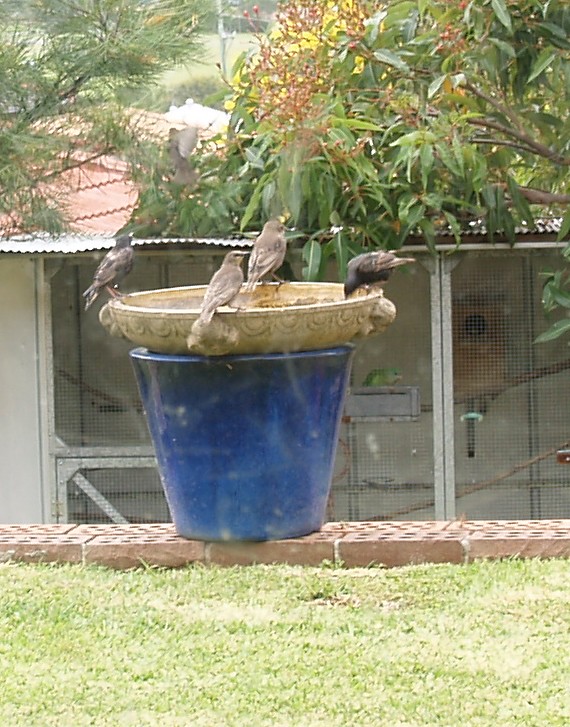This daytime outdoor color photograph features a charming DIY birdbath setup in a yard. In the foreground, lush green grass leads up to a small brick ledge. Positioned on this ledge is a substantial blue planter pot, which serves as a base for a homemade birdbath. The birdbath itself contains food instead of water and is surrounded by four birds. The birds at the left and right are darker in color, while those at the front and back are lighter gray. One of the darker birds is dipping its beak into the birdbath. In the background, a variety of plants, including a pine tree and berry bushes, enhance the natural setting. Also visible is a birdcage containing a green bird and a birdhouse with a hole, set against the backdrop of a structure's roof peeking from the left side of the image. The scene suggests an overcast day, with diffused sunlight adding a soft touch to the vibrant nature display.